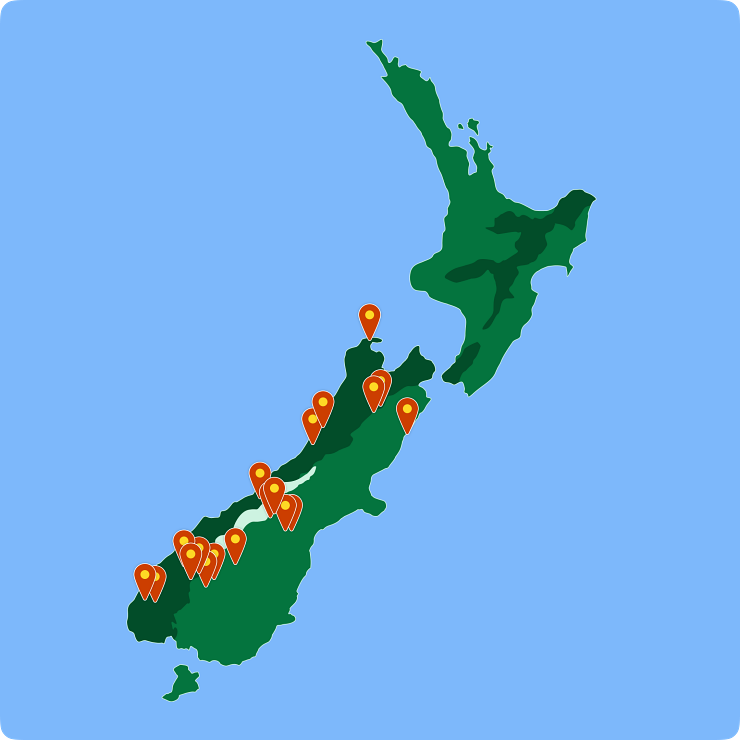This detailed map image of New Zealand features both the North and South Islands amidst a blue ocean background, emphasizing their distinct separation. The islands are depicted in varying shades of green, with the left coast of the South Island appearing darker and patches of lighter green scattered in the middle, suggesting topographic elevation differences. The map is a computer-generated graphic without any text or labels. The South Island is marked by multiple pinpoints, which are red teardrops with yellow circles in the center, primarily concentrated on the left side. These pinpoints, numbering around twenty, could indicate significant locations or events, though the map offers no specific context or legends. Additionally, a small strip of white is visible on the South Island, adding to the map's intricate detail. The map is devoid of any textual information, relying solely on visual cues.